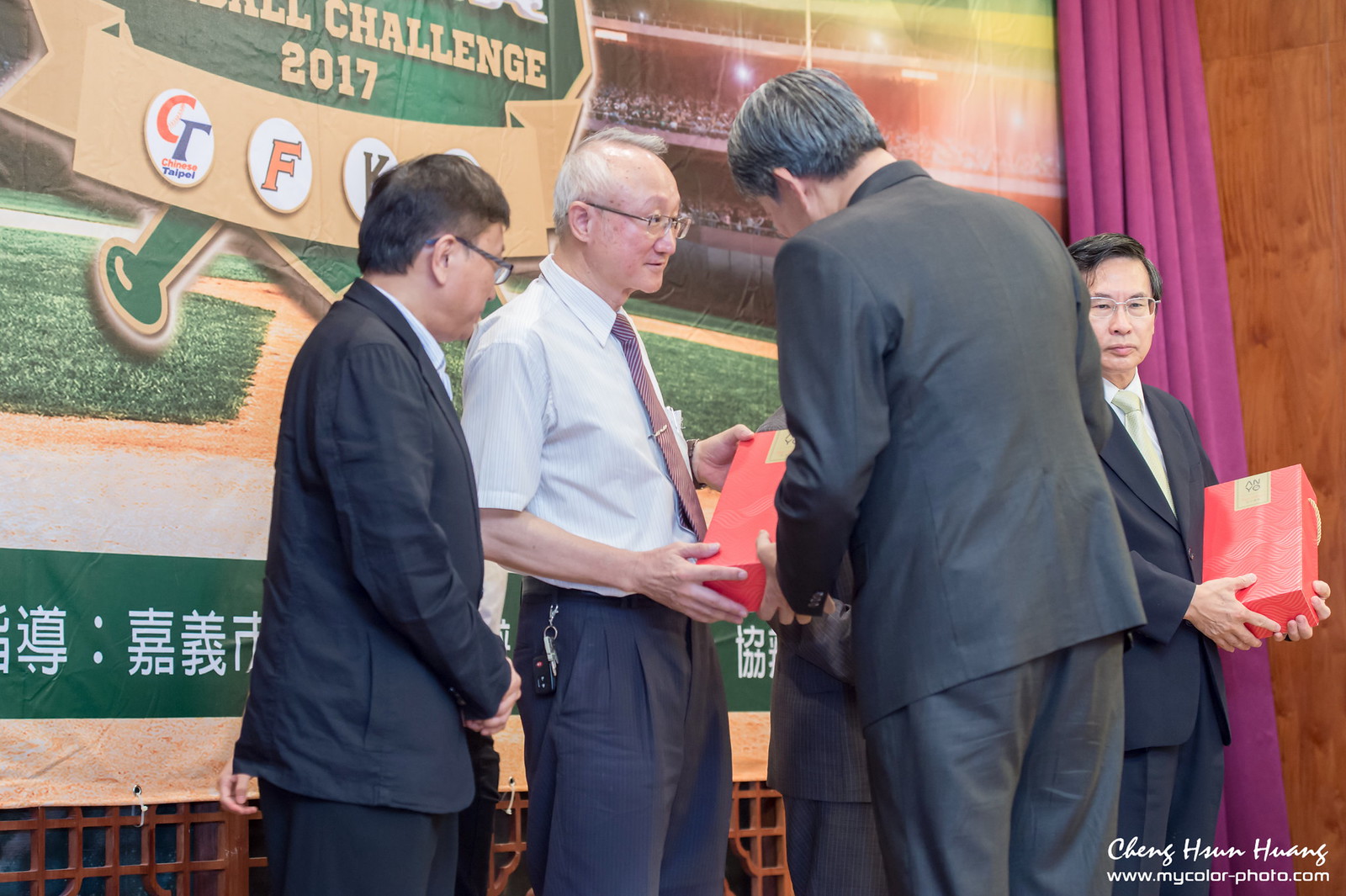In this photograph, there are five individuals prominently featured, with most of them dressed in black coats and pants, exuding a formal atmosphere. Notably, one man breaks the uniformity by donning a shirt, pants, and a tie. He is engaged in handing over a red-colored box to another man whose back faces the camera, adding an element of intrigue to the exchange. Additionally, another individual is seen holding an identical red box, suggesting a ceremonial or award-giving event. The backdrop features a large board with an image of a stadium and partially readable text, hinting at a sports-related theme. To the right of the board, a pink curtain adds a splash of color, juxtaposed against a brown wooden wall. The bottom right corner of the image contains the text "Cheng Huan Huang, www.mycolor-photo.com," indicating the photographer and their website.